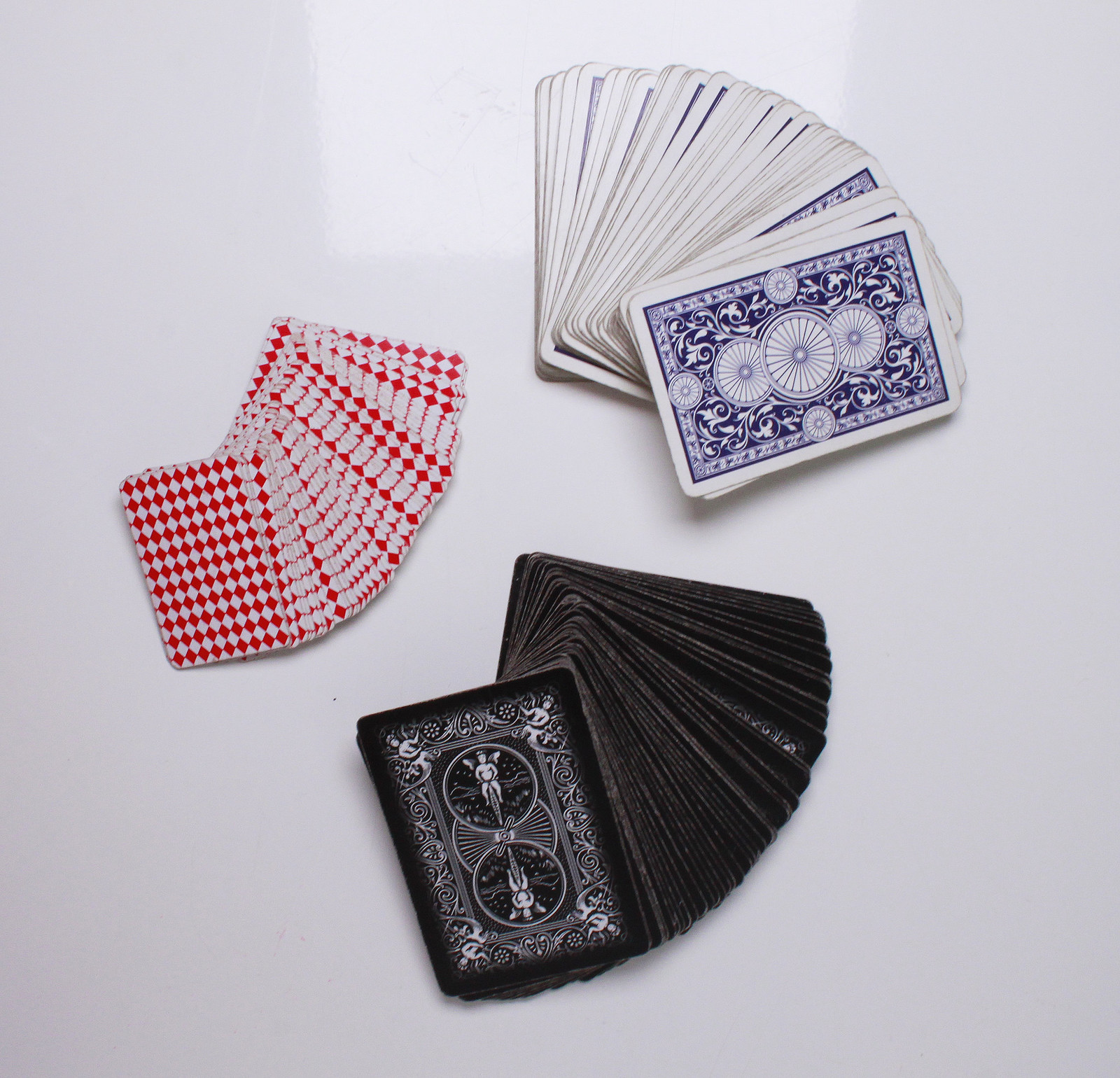This square-format photograph showcases three distinct decks of playing cards meticulously arranged on a pristine white surface. A slightly brighter white shadow in a square shape is noticeable at the top center, adding a subtle highlight to the composition. The decks are separated into three individual stacks, each fanned out in a unique direction, enhancing the visual appeal.

The upper right deck exhibits a calming blue color palette. Each card has a white background with a striking blue center adorned with a series of three circles, the largest one in the middle. Running vertically from the bottom to the top of each card is an intricate floral pattern.

At the lower center of the image lies a black deck, fanned out towards the lower right. These cards feature a bold black border encasing a refined white design. The centerpiece showcases two angelic figures riding a bicycle, arranged vertically with one figure on top of the other, exemplifying intricate artistry.

To the left, a red deck of cards is fanned out towards the right with a slight downward angle. The back of each card features a vivid red and white diamond pattern, adding a traditional yet striking visual contrast to the overall arrangement.

This carefully composed photograph not only highlights the unique design elements of each deck but also showcases the artful arrangement and the elegant simplicity of the white background.